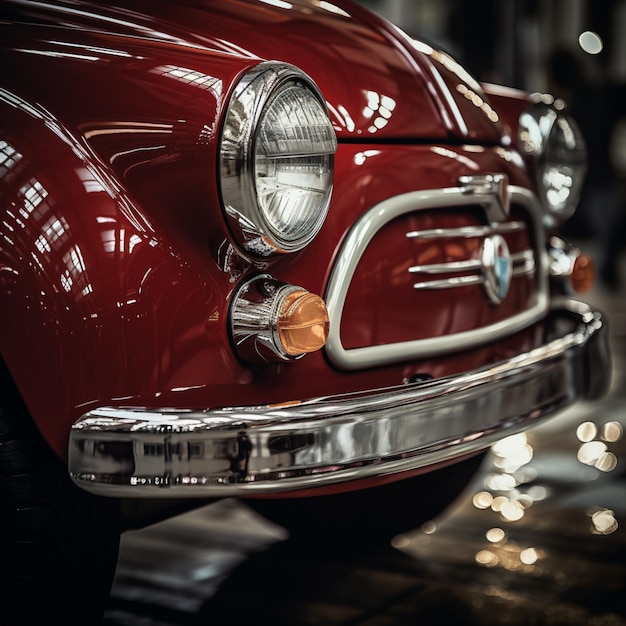This photograph captures an extreme close-up of the glossy front end of a vintage sedan, likely from the 1940s or 1950s, under city lights at night. The car, a deep, candy-apple red, gleams as it reflects surrounding streets and windows. The chrome bumper, which shines brilliantly, frames the lower part of the image. Above the bumper, a red and blue logo sits within a curved rectangular frame on the sloped hood. Flanking this logo are the car’s silver headlights and smaller amber turn lights. The chrome grill adds an additional element of shine to the front facade. Although the main focus is the pristine car front, hints of the out-of-focus wheels and indistinguishable lights can be seen towards the bottom and top right corners of the image.